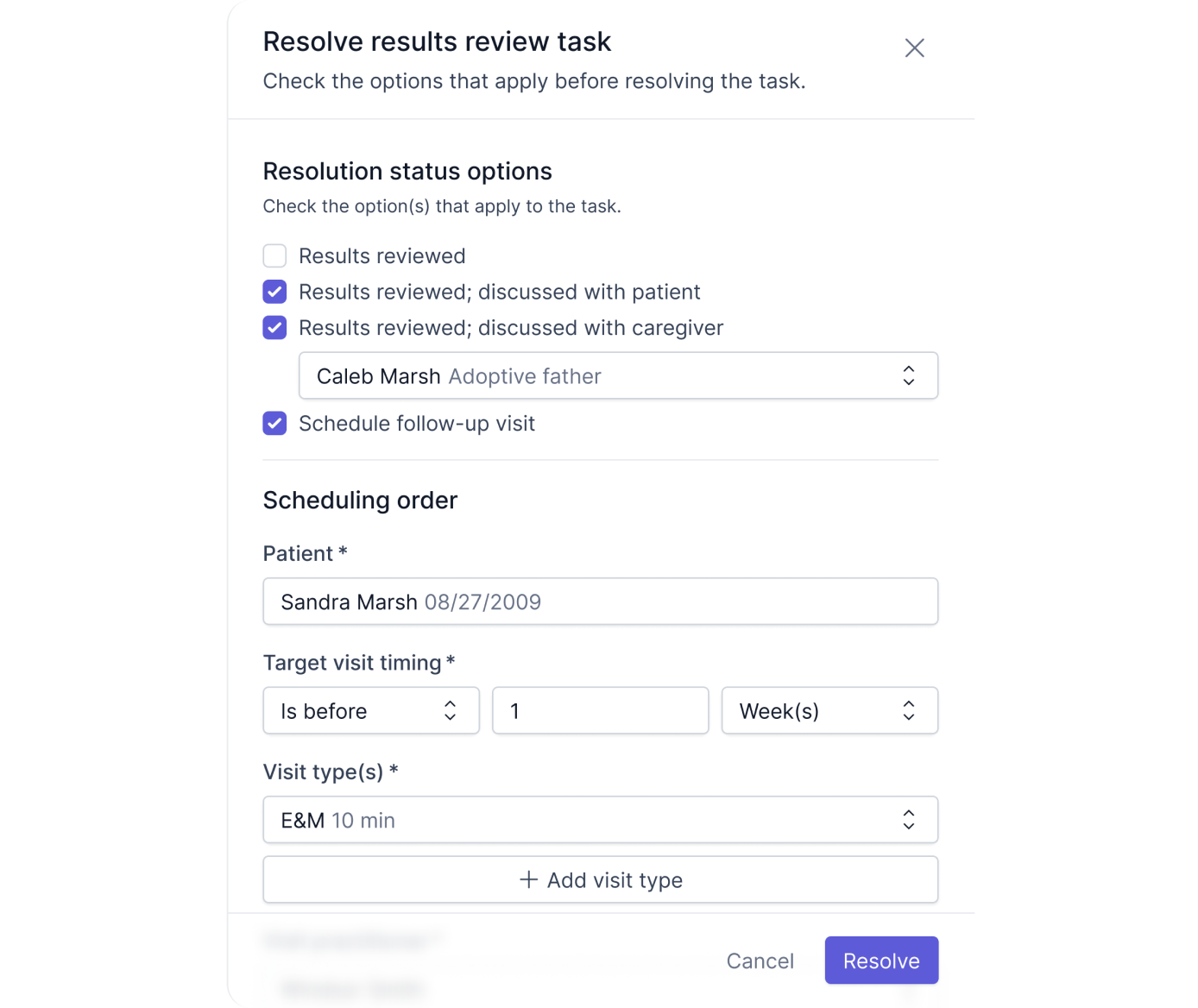The image depicts a section of a task resolution interface related to patient management. At the top, the header "Resolve Results Review Task" is prominently displayed in bold black letters. Below, there is a prompt instructing users to "Check the options that apply before resolving the task." 

Another section is titled "Resolution Status Options" and provides choices for the user to select: "Results Reviewed," "Results Reviewed Discussed with Patient," and "Results Reviewed Discussed with Caregiver."

Under the "Patient Information" section, the name "Caleb Marsh" appears with the designation "Adoptive Father." A drop-down menu allows users to select the relationship, and purple checkboxes indicate selected options, such as "Schedule Follow-up Visit."

Next, the "Scheduling Order" section, marked with an asterisk to indicate required fields, requests the patient's name, "Sarah Marsh." The "Target Visiting Timing" field, also marked by an asterisk and highlighted in orange, shows "1" week(s) from the current date. Users can choose the length of time through a drop-down menu.

The "Visit Type" field, marked with an asterisk, lists "E&M 10 minutes," with an option to select different visit types via a drop-down menu. There is also a white space outlined with dotted lines for adding "Additional Visit Type."

At the bottom of the interface, two buttons are visible: "Cancel" and "Resolve Task," the latter highlighted in purple.

The overall image relates to the management of patient follow-ups, involving coordination between doctors, patients, and potential caregivers.